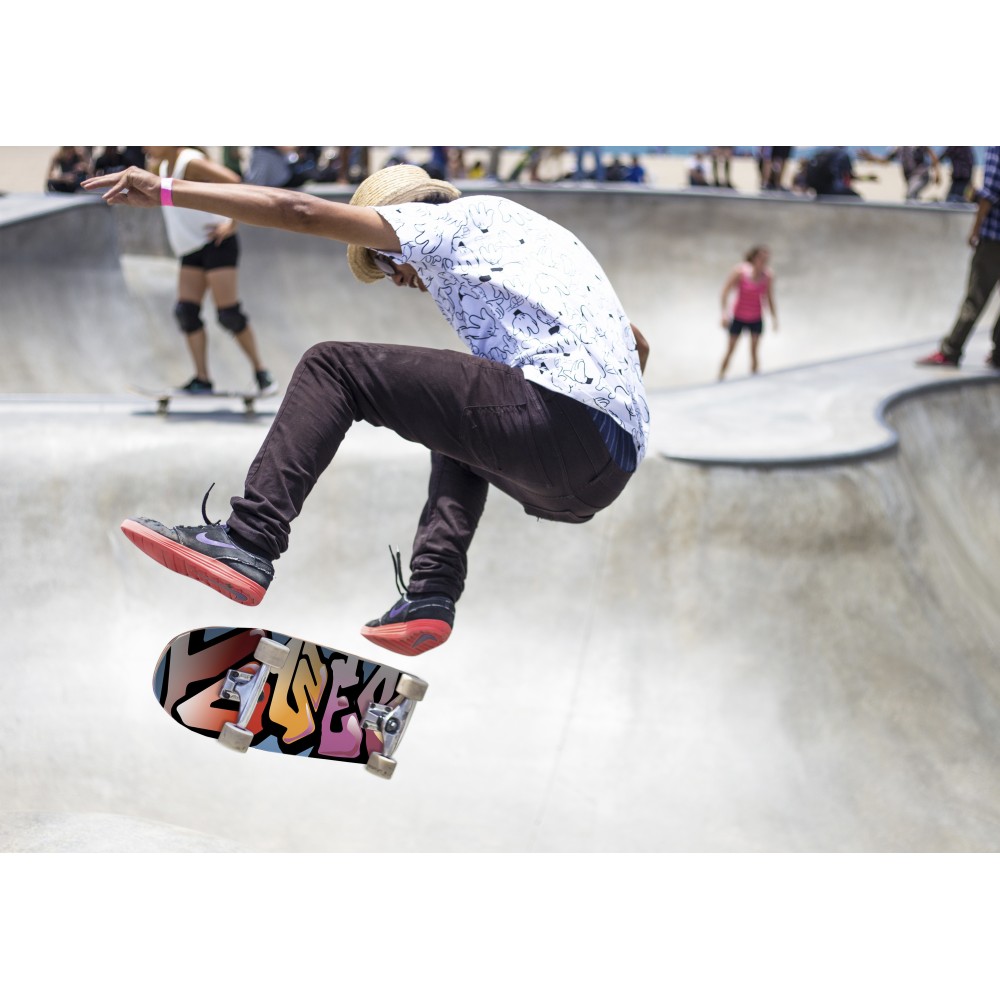In this dynamic photograph of a skate park, a man is captured mid-air performing a kickflip on his skateboard. The central figure of the image, he wears black jeans, black and red sneakers featuring a red sole, and a white short-sleeve t-shirt adorned with black doodles. His outfit is topped off with a light gold straw hat and a pink wristband on his left wrist, which is extended for balance. His skateboard, vivid with graffiti artwork in blue, pink, yellow, and red, and equipped with white wheels, is prominently beneath his feet. The background reveals a typical skate park setting with concrete ramps in gray tones. Several other skateboarders populate the scene: one woman in a pink shirt and black shorts, another in a white tank top, black shorts, and black knee pads, and a third person in a blue shirt with black jeans and red shoes. The composition effectively captures the energy and diversity of the skate park environment.